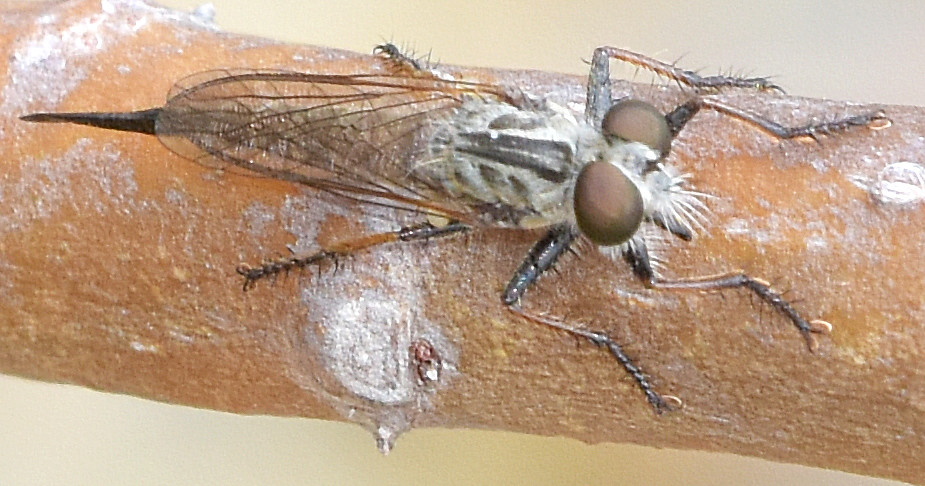This detailed, close-up image captures a robber fly, specifically the Ephyria astuans species, resting on a brown twig scattered with white patches of mold or dust. The fly is perched from a left to right orientation. Its prominent features include two large brown, bulbous eyes atop its head. The insect's thorax is white with streaks and stripes, capped with transparent wings folded on its back. The fly's elongated body tapers to a pointed end, recognizable as the distinctive pointed tail typical of the species. Whitish fur-like feelers protrude from its head, giving it a bearded appearance. Its six hairy legs, equipped with gripping, fang-like extremities, secure its hold on the twig. This remarkable close-up highlights the unique and detailed anatomy of the robber fly, emphasizing its characteristic winged structure and pointed body.